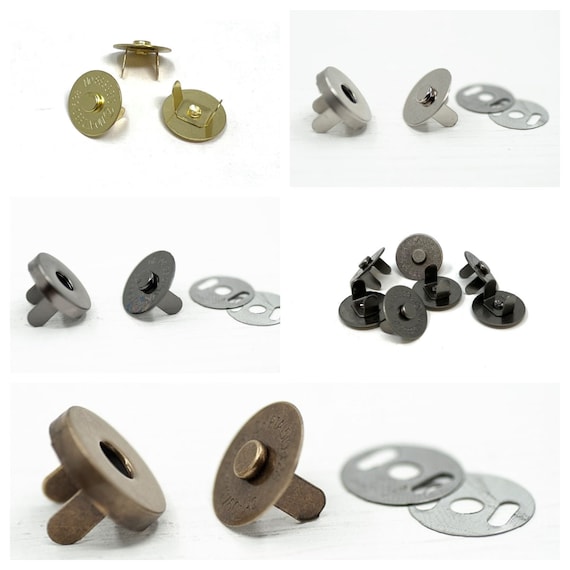The image is a square collage, approximately four inches high by four inches wide, showcasing various types of metal fasteners in a professional studio lighting setting. The collage is divided into six smaller photos arranged in two columns, each containing three rows.

In the upper left-hand corner, three small, light gold discs with a raised center resemble the inside of a snap. To their right, on a light gray background, are two silver circles: one with a central hole flanked by push tabs on the backside, the other featuring a raised center with similar push tabs. Further right are two small silver discs, each with a central hole and oval holes flanking the center hole.

The middle row features the same configuration as the upper right but depicted in a lighter gray and more grayish tone. To the right of this, a set of plain black discs with a raised central area has push tabs on the back.

The bottom row extends across the entire width of the collage, showing various fasteners. On the left are large brown discs: the leftmost has a central hole with two back tabs, and the right one has a raised center also with back tabs. On the far right, two silver discs with central holes are each flanked by additional oval-shaped holes.

The materials and colors vary across the photos, including brass, silver, black, and brown, indicating a collection of different types of fasteners possibly used in various applications. This detailed professional product photography suggests usage intended for e-commerce displays, with minimal reflections indicating high-quality studio lighting.